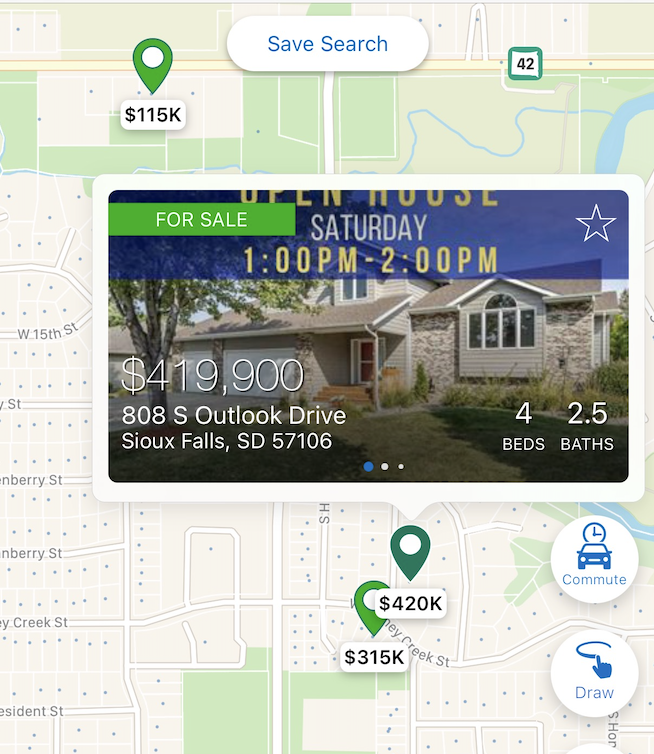A detailed map is displayed, featuring green arrows that pinpoint specific locations. One prominent arrow is marked with "115K" inside a white circle, while another similarly colored arrow indicates "315K" at a different location. Nearby, a slightly different shade of green denotes the area marked "425 to 420K," likely indicating a selected item. Adjacent to the map is a tile showing a front view of a house from the driveway with the caption, "Open House Saturday 1 p.m. to 2 p.m." This two-story house is listed for sale at $419,900, featuring four bedrooms and two and a half bathrooms, located at 808 South Outlook Drive in Sioux Falls, South Dakota, 57106. The tile includes three photos, with the first one currently displayed. A green banner reading "For Sale" spans part of the image, and there's a star icon allowing users to favorite the listing. Additionally, there are buttons labeled "Commute" and "Draw" for user interaction.